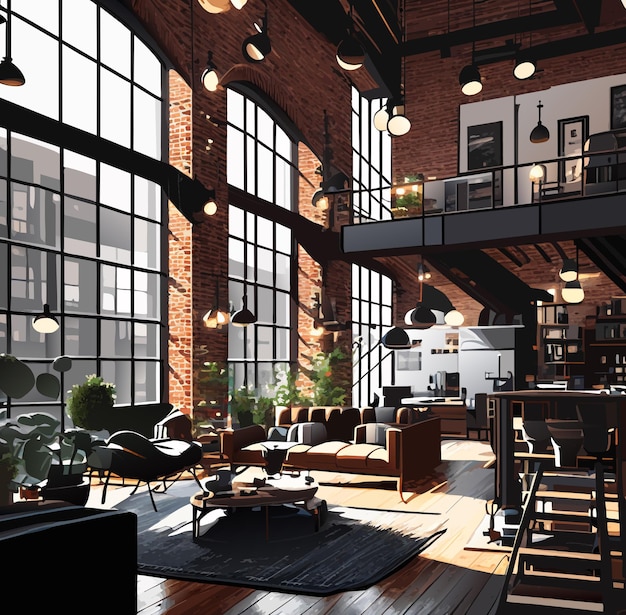This square-shaped image depicts a luxurious lofted apartment, likely a converted old factory or warehouse, situated in a metropolitan area. The apartment boasts very tall ceilings, reaching approximately 40 feet, emphasizing the loft's spacious and airy design. The walls are adorned with classic red brick, adding a rustic charm, while the enormous plate glass windows, framed with black crisscrossing frames, flood the space with natural light and offer a light gray cityscape view.

The ground floor showcases a modern living area furnished with a long brown couch and complemented by a blue rug, alongside a modern chair and several plants. The flooring is light brown hardwood, creating a warm and inviting atmosphere. The presence of a black rug and black pendant-style lights hanging from long poles contribute to the loft's warm industrial aesthetic. The kitchen, located behind the living area, features sleek, modern appliances including a steel refrigerator, large stove, microwave, coffee pot, and a breakfast center island. This area also includes stools for casual dining.

An industrial-style black staircase with black edges ascends to the open second story, which overlooks the living area below. This upper level is equally well-appointed with an entertainment table, modern furnishings, and additional pendant-style lights. The black light fixtures, both on the ground floor and upstairs, are suspended from long poles and are fitted with black covers and warm yellow light bulbs, enhancing the loft's modern-industrial vibe. Overall, the loft is a harmonious blend of modern luxury and industrial charm.